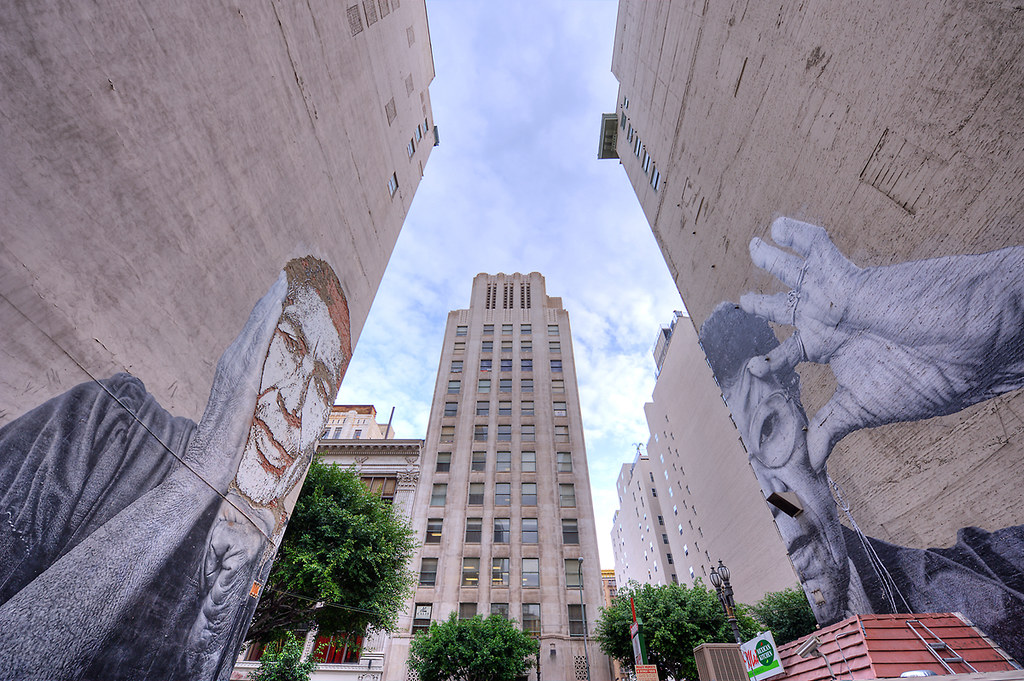The image depicts a vibrant downtown area under a clear blue sky adorned with fluffy white clouds. Dominating the skyline are several towering buildings, two of which feature large, striking murals. On the left, a mural of former President Barack Obama captures his likeness vividly; he is wearing a suit, appears cheerful, and has his hand raised beside his face. On the right, another mural portrays an Asian man with dark hair and small, round glasses. He is dressed in a black suit and holds his thumb and forefinger to his eye, seemingly holding it open, with a small black emblem positioned at the end of his nose. These artworks add a unique and artistic flair to the urban landscape.